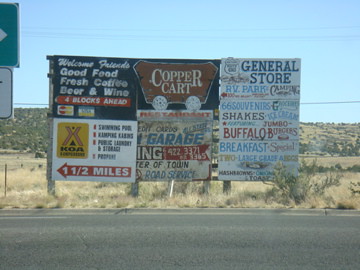In this outdoor image, a cluster of signs is prominently featured on the side of a roadway. The road in the foreground is asphalt with a faded white line at its edge, winding horizontally. Directly behind the signs, the ground is covered in dry, scraggly grass and bushes, giving the area a desert-like feel.

The signs, mounted together on a large board, offer a variety of messages. They include a blue and white sign welcoming friends with promises of good food, fresh coffee, beer, and wine. Adjacent to it is a black and copper-colored sign for the Copper Cart. Another sign directs to a KOA campsite located one and a half miles ahead, indicated by a red arrow.

Additional signs advertise a general store, RV park, camping facilities, and a restaurant and garage named Cardo Garage. There is also a sign for 66 Souvenirs, promoting shakes, buffalo jumbo burgers, and a breakfast special. 

In the background, a gently sloping hill covered in desert brush stretches out, with some scattered green patches. Above, the sky is a clear medium blue, traversed by power lines that slope slightly downward, linking unseen poles outside the frame. A small green and white sign and a white and black sign are also visible near the top left corner of the image.